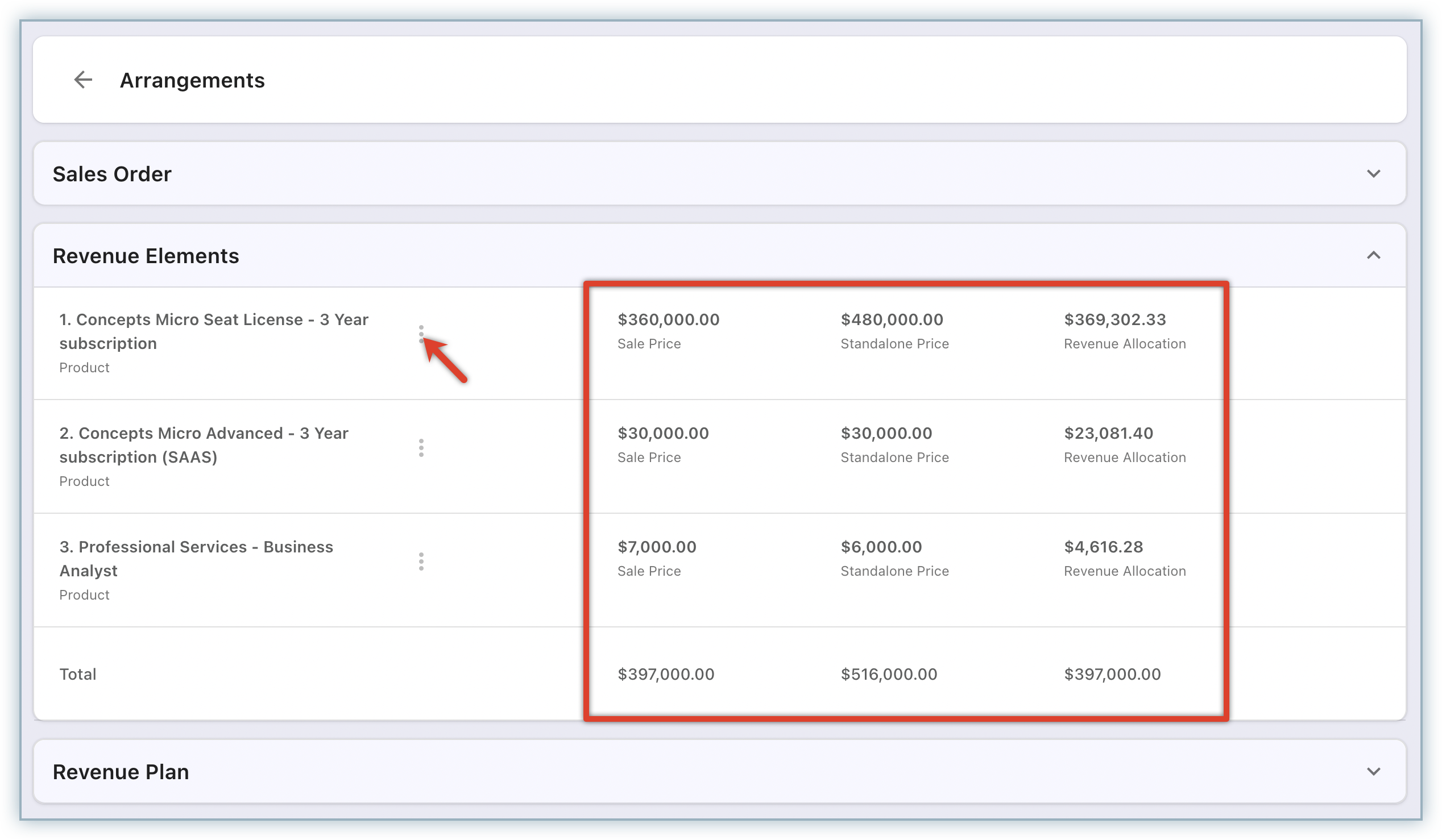The screenshot displays a financial interface with detailed revenue information. At the top, a title labeled "Arrangements" is seen alongside a left-pointing arrow for navigating back to the previous page. Directly below the title, the section "Sales Order" is indicated, followed by "Revenue Elements," which lists three distinct entries.

1. **Concepts, Micro, Seat License, 3-Year Subscription**
    - Subsection: Product

2. **Concepts, Micro, Advanced, 3-Year Subscription, SAS**
    - Subsection: Product

3. **Professional Services, Business Analyst**
    - Subsection: Product

For each of these entries, three different prices are outlined horizontally:
- Sale Price
- Standalone Price
- Revenue Allocation

A total at the bottom aggregates these prices for all three entries.

At the bottom of the interface, there's a section labeled "Revenue Plan" which can be expanded, similar to the "Sales Order" and "Revenue Elements" sections, both of which feature expandable arrows. The "Revenue Elements" section is currently expanded, revealing all the detailed pricing information mentioned above.

Additionally, a red box highlights the revenue figures, and a red arrow points to a menu represented by three dots next to the first entry: "Concepts, Micro, Seat License, 3-Year Subscription." This highlights a specific action or option related to this entry.

Overall, the interface appears straightforward, with clearly delineated sections and expandable menus for detailed views.